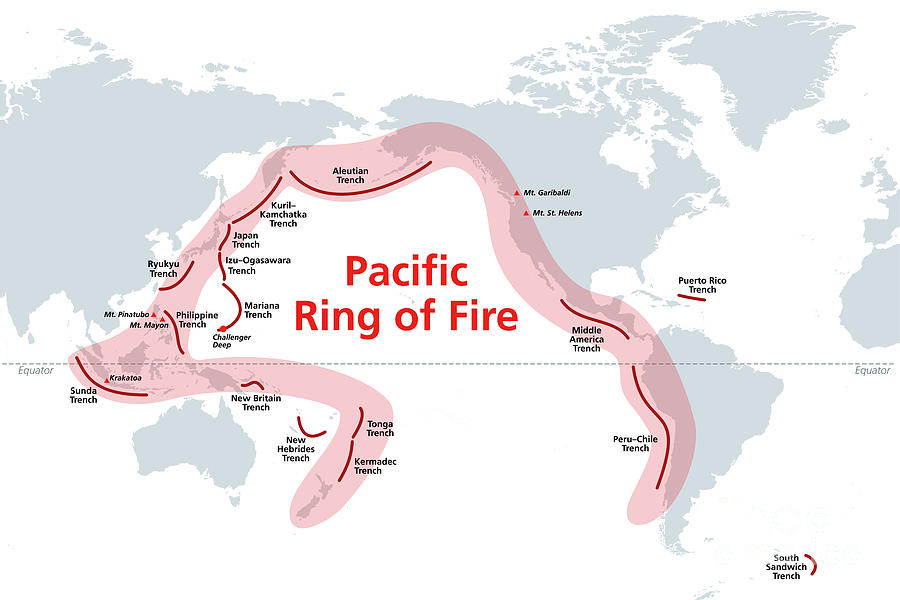This is a detailed map depicting the Pacific Ring of Fire, set against a white background with continents shaded in light blue. The central feature is a slightly opaque pink border that traces a path from the southern tip of South America, along the western coastlines of North and South America, across the Bering Strait, down the eastern edge of Asia, and around the eastern side of Australia. Prominently displayed in bold red letters across the middle of the map is the title "Pacific Ring of Fire." The pink-bordered area highlights various geographical features and trenches associated with the Pacific Ring of Fire, including notable ones such as the Peru-Chile Trench, Middle America Trench, Puerto Rico Trench, Aleutian Trench, Japan Trench, Izanagi Trench, Ryukyu Trench, Sunda Trench, New Britain Trench, New Hebrides Trench, Tonga Trench, and Kermadec Trench. Additionally, the map includes the names of key volcanic mountains like Mount St. Helens and Mount Gibraltar. The presence of these geographical features underscores the seismic and volcanic activity characteristic of the Pacific Ring of Fire.